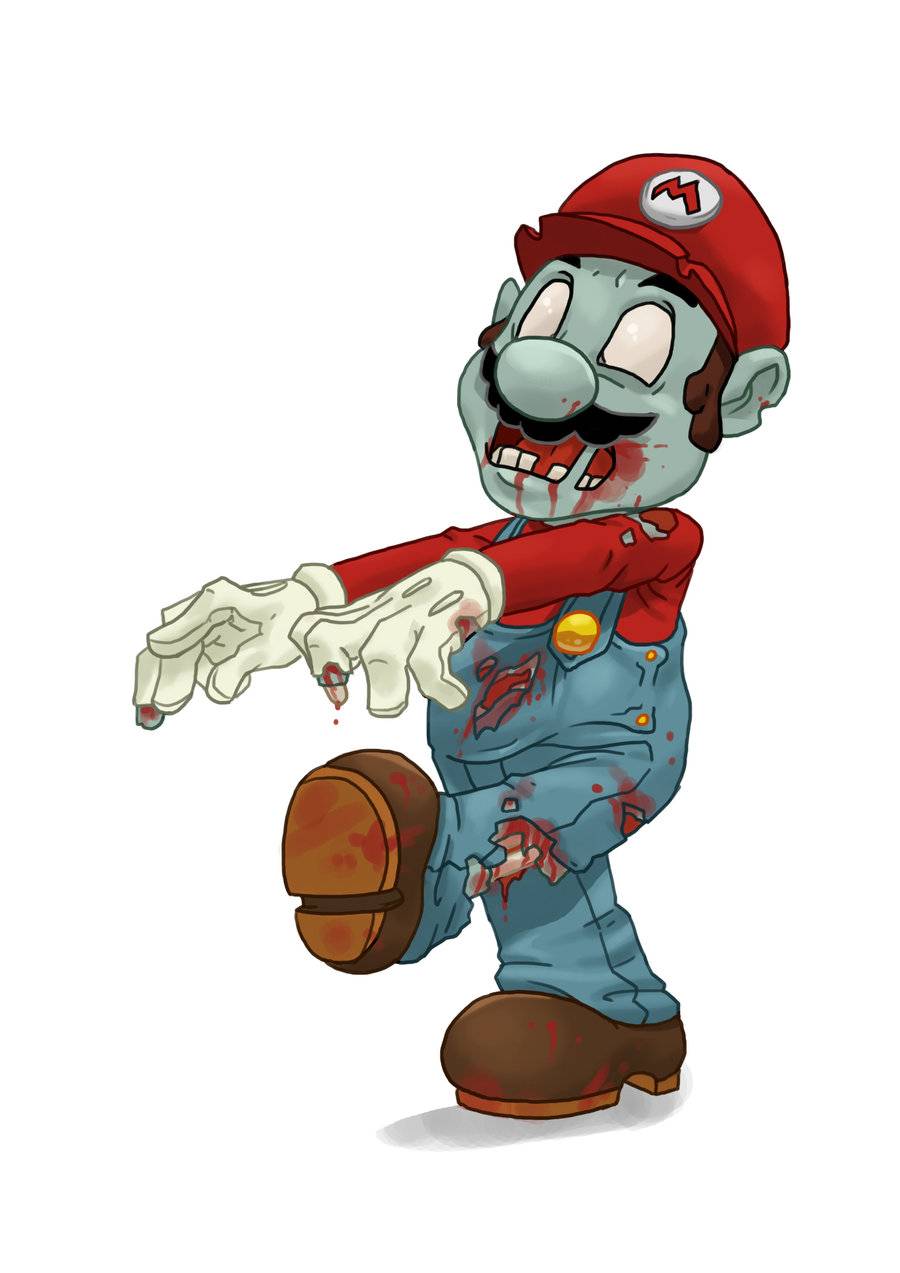This detailed illustration depicts a zombie version of the iconic video game character Mario. Retaining all his recognizable traits, Mario sports his traditional red cap with a white circle featuring a red 'M', a matching red shirt, blue overalls with gold buttons where the straps meet the overalls, white gloves, and cartoonish brown shoes. However, his usual cheerful demeanor is replaced by a ghastly visage. Mario's face is a pale, grayish-teal color, with eyes turned into pure white voids devoid of pupils or irises. His trademark mustache and brown sideburns are still present, but his mouth is missing teeth and is smeared with blood which also stains his gloves. The overalls are tattered, revealing missing chunks of flesh and a bone exposed beneath a rotting pant leg. Mario's overall appearance is ghastly, with bits of muscle and skin missing, creating a terrifying, rotting effect. He is depicted in a classic zombie pose, with his arms outstretched in front, and one leg extended in a stiff, straight gait.